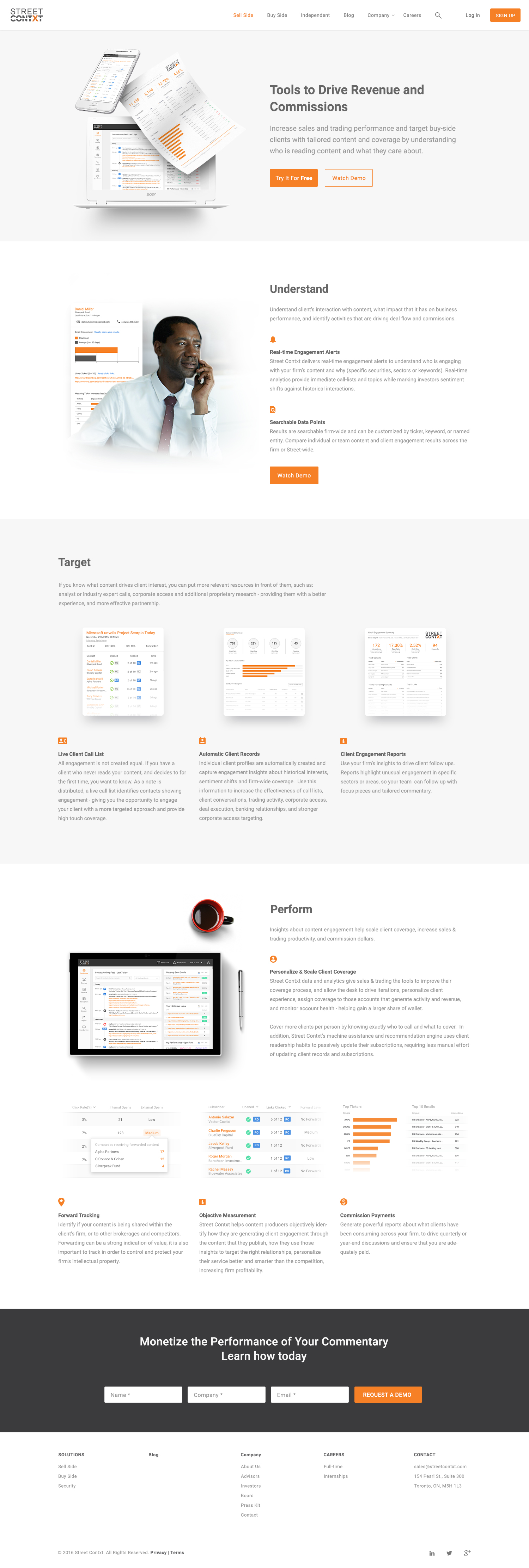The image is a tall, portrait-oriented screenshot of an app or web page, approximately three times as tall as it is wide. At the very top, there is a white bar with a header in the left corner reading "Street," followed by text that is too small to discern clearly but ends with a red or orange letter. To the right of this header, there are several sub-headers or clickable links, the first of which is highlighted in orange, followed by an orange rectangular box with white lettering.

Below this section, there is a long, rectangular gray border that contains the text "Tools to Drive Revenue and Commissions." It features a laptop, a phone above it, and a paper nearby, flanked by two boxes—one orange and one white.

Further down, a white border displays the word "Understand" alongside an image of a man in a suit and tie, appearing deep in thought with a graph behind him. Under this, a gray box labeled "Target" contains several paragraphs of text and three evenly spaced pieces of paper, each with a description underneath.

Next, the word "Perform" is presented next to a red and black object and an iPad with a pen, showcasing several charts. Below, more charts are displayed.

At the very bottom, the text "Monetize the Performance of Your Commentary" invites viewers to "Learn How Today" and provides fields for signup information, concluding with an orange box with white lettering for submission.